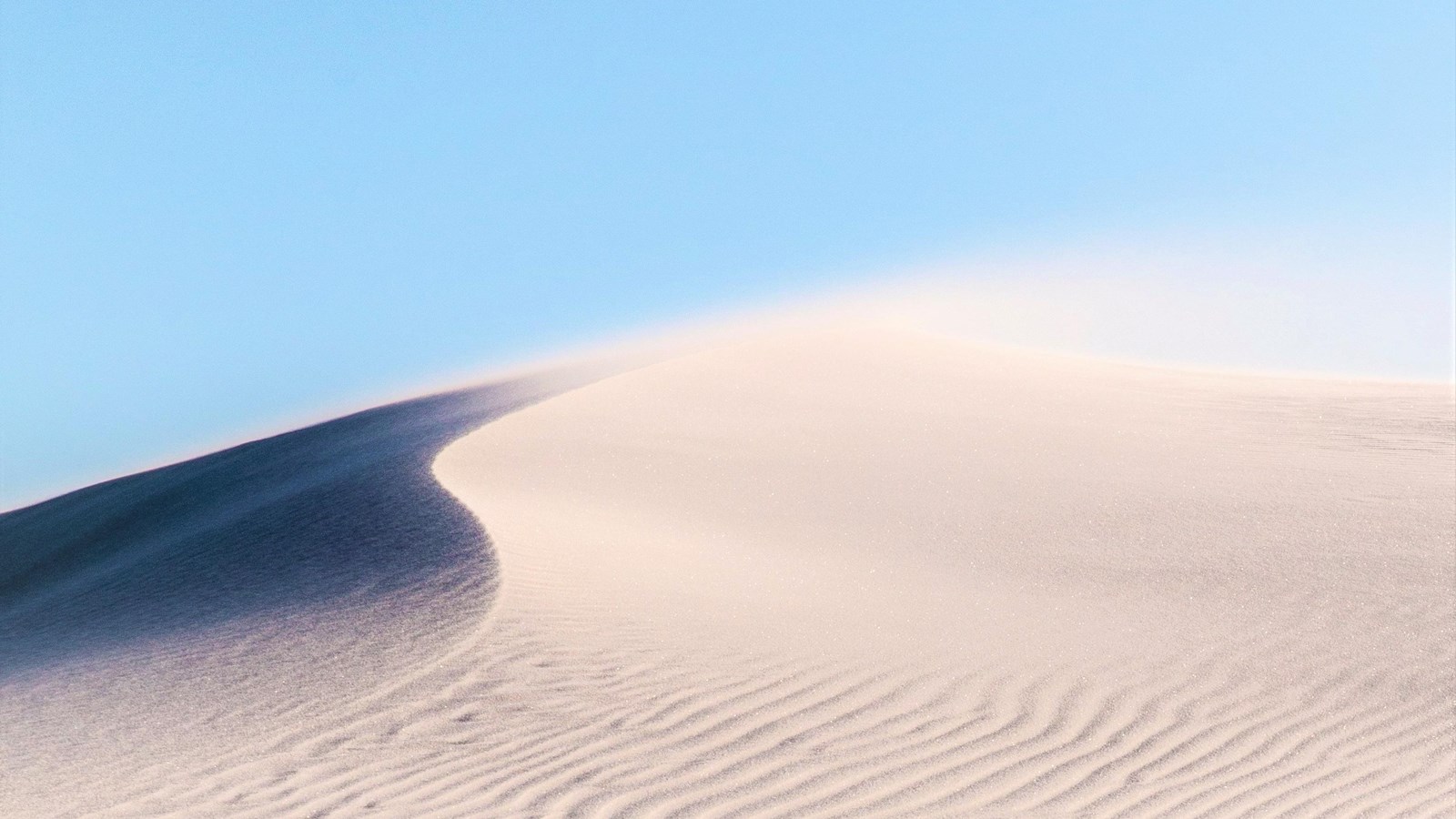This image depicts a striking desert sand dune under a clear blue sky, devoid of any clouds. The scene illustrates a white sandy expanse with varying textures—ripples of sand running off to the right in the foreground and smoother textures further back. At the crest of the dune, particles of sand are visibly being blown by the wind, creating a misty effect against the horizon. The wind appears to be blowing from left to right, evidenced by the small particles of sand suspended in the air. The left side of the dune is cast in deep shadow, indicating that the sun is positioned to the right, casting detailed contours and ridges along the dune. These ridges run from the middle of the image, curving gently down to the bottom right. The bottom left corner of the picture exhibits darker shadows that gradually blend into the lighter sand as the eye moves toward the center. This combination of light, shadow, and wind-blown sand captures the dynamic and serene essence of the desert landscape.